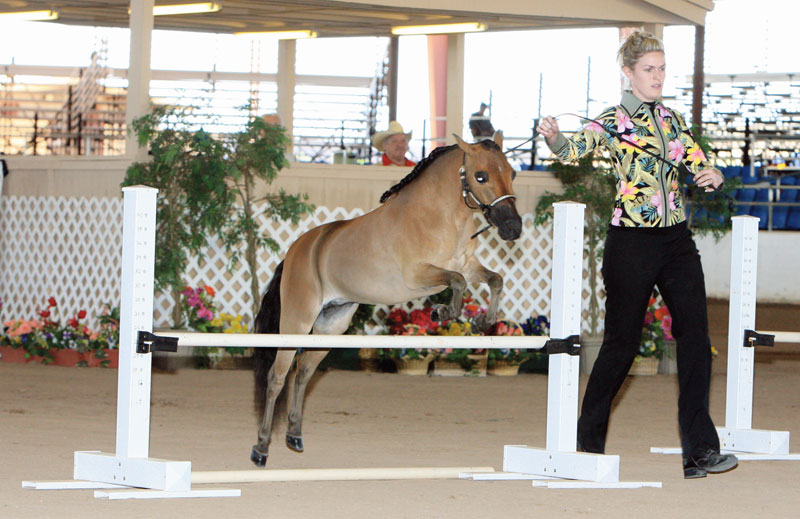This photograph captures a captivating moment at a horse show featuring a small, light brown miniature horse, or pony, in mid-jump over a white bar held by two white wooden stands, indicative of an equestrian obstacle. The pony, in an impressive leap with its front legs raised and back legs still on the ground, showcases its agility and grace. Its distinguished black mane, tail, and gray snout and eyes enhance its striking appearance. 

Leading the pony is a woman, guiding it with a leash attached to its harness. She is dressed in black pants, boots, and a colorful flowery shirt, her blonde hair neatly piled on top of her head. She holds the reins high, seemingly assisting the pony's jump. 

In the background, a man sporting a cowboy hat stands or sits, observing the scene, with hints of stadium seating visible on the right side, suggesting an outdoor competition setting. A small tree with green leaves and a latticework fence adorned with plants add to the picturesque nature of the event.